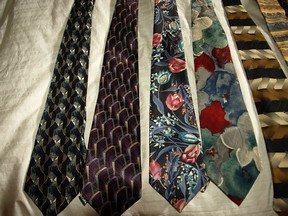The image displays six men's ties meticulously laid out side-by-side on a white quilted bedspread, with the tips just overlapping the edge. Each tie features a distinct design and color scheme, creating a rich tapestry of patterns. The first tie showcases a black and white squiggly pattern with a white end. Moving to the right, the second tie features a purple design with a silver line and a scale-like pattern. The third tie presents a classic floral motif with blue, pink, and light green flowers set against a light backdrop. The fourth tie also displays a floral theme but with more abstract white, red, and green flowers. Next is a tie with a traditional checkered pattern in off-white, brown, tan, and black, accented with stripes. The last tie in the frame, only partially visible, appears to be goldish-blue and striped. The arrangement suggests that someone is carefully selecting a tie for the day.